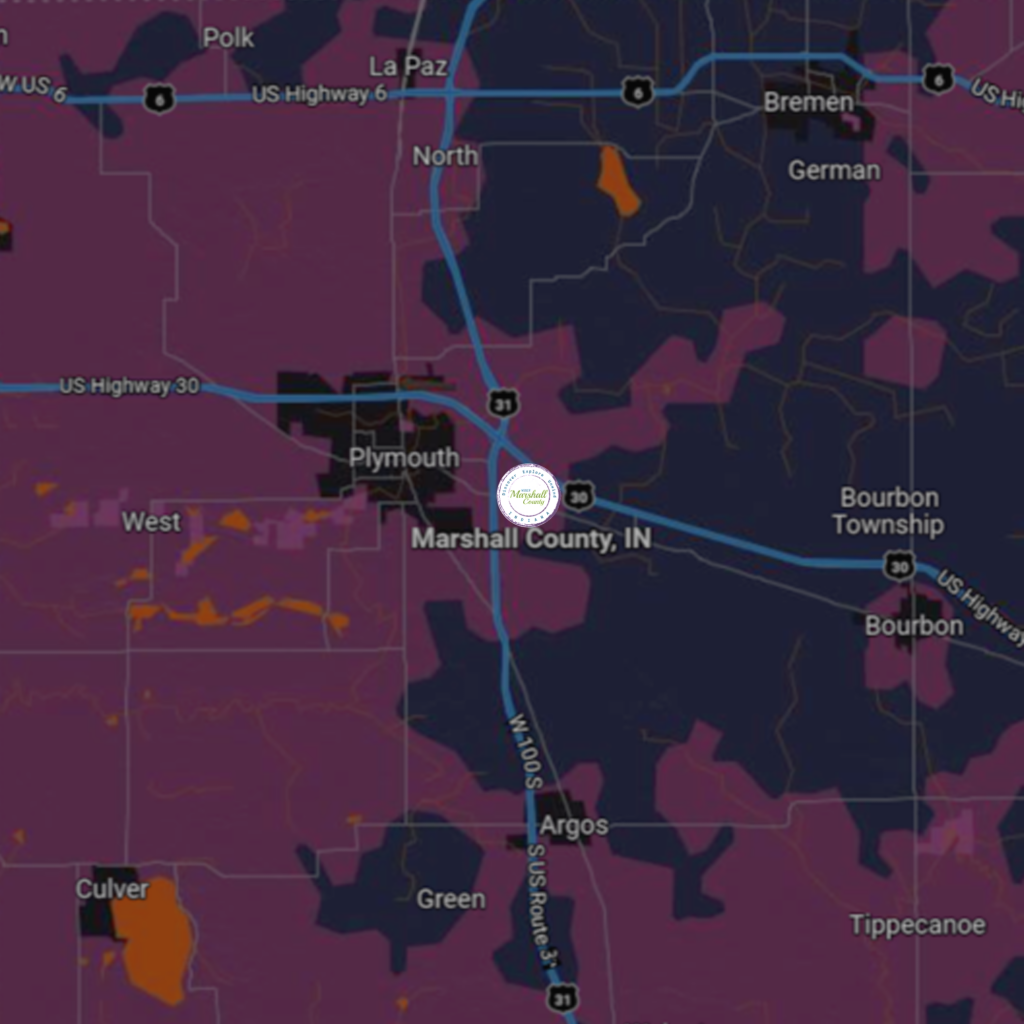This image captures a detailed and colorful map with various notable features and landmarks. The land area is highlighted in purple, while the water areas add a blue contrast. Starting from the left corner of the map, approximately an inch inward, there's a distinct border of land resembling shoulders and a neck with a head extending toward the top right. Adjacent to this, another smaller landmass extends off the top. About an inch further to the right, a larger landform stretches down around three inches, then arcs to the right, back left slightly, drops down a bit, turns left again, passes halfway down, and extends further left. This landmass forms a pronounced peninsula about an inch wide, stretching an inch down and then extending off to the right side.

Along the top edge of the map, approximately an inch from the border, a blue line is marked as Highway 6. Another notable feature is a line running vertically from the center all the way down, labeled W100S US Route. Prominently in the center is a white circle with indecipherable text surrounded by the caption "Marshall County IN." Midway across the map, there is a diagonal label reading "USA Highway 30."

In the bottom left corner, roughly two inches inward, an orange spot approximately two inches long and an inch wide is marked with the word "Culver" in white text. The lower right corner features the label "TIPPECANOE," positioned just right of an interstate mark. On the left side, the word "Green" is displayed. Various towns like Plymouth, German, Bremen, and North are also prominently listed, helping to orient the viewer within the region depicted.